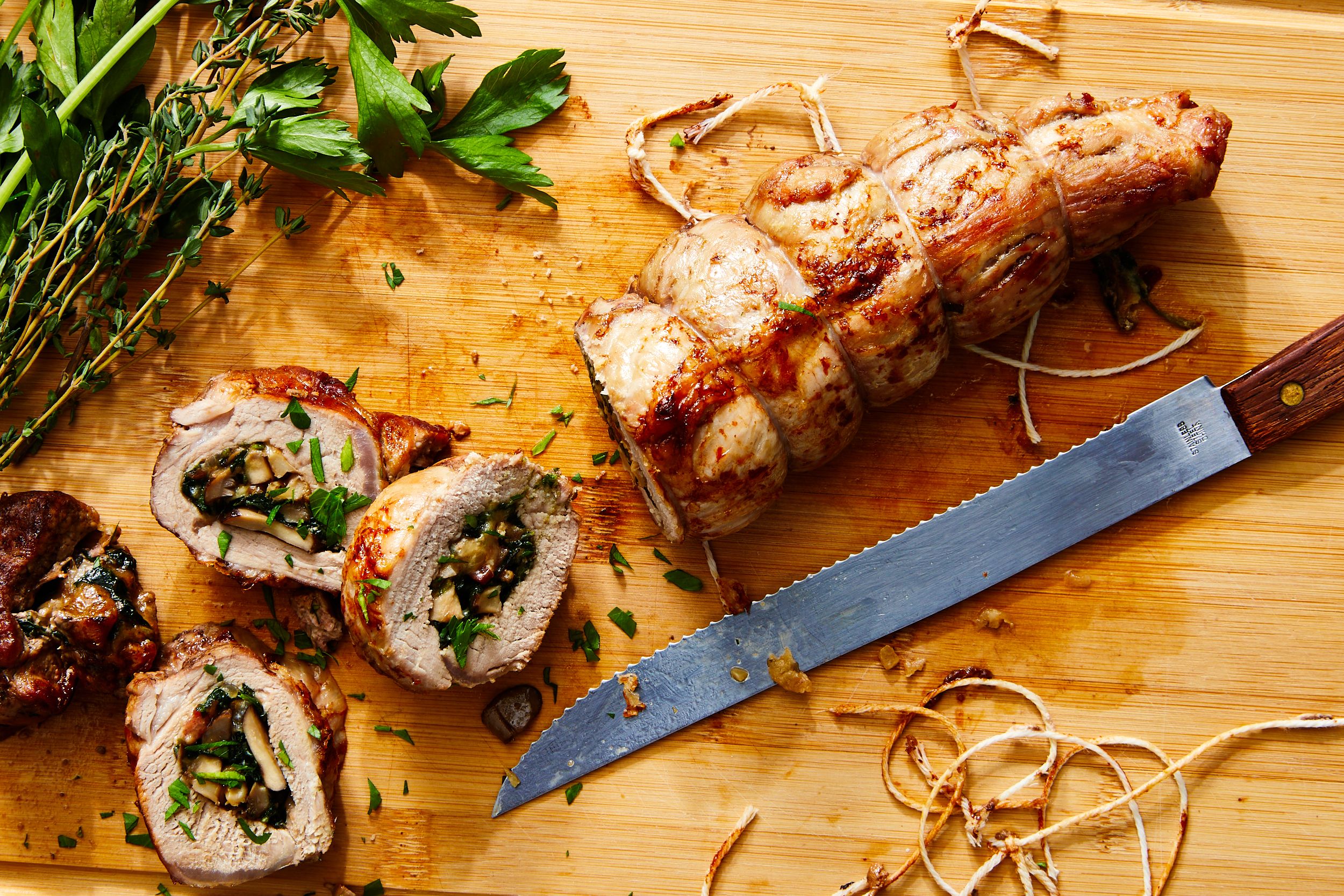The image displays a beautifully prepared, long log of white meat, likely chicken or pork, around 12 inches in length, resting elegantly on a cutting board. The meat has been expertly rolled up, stuffed with a flavorful mixture of herbs, mushrooms, and perhaps garlic and thyme, then tied together with string before being baked or grilled to perfection. The exterior of the meat features a mouthwatering light brown, caramelized finish. Four succulent slices have already been cut from the roll, revealing the delicious stuffing within. Scattered around the cutting board are green herbs, possibly parsley, and remnants of cut string. A serrated knife with its blade facing up lies to the right of the meat, ready for further slicing and serving. The overall scene suggests a dish that is not only visually appealing but also delectable and ready to enjoy.